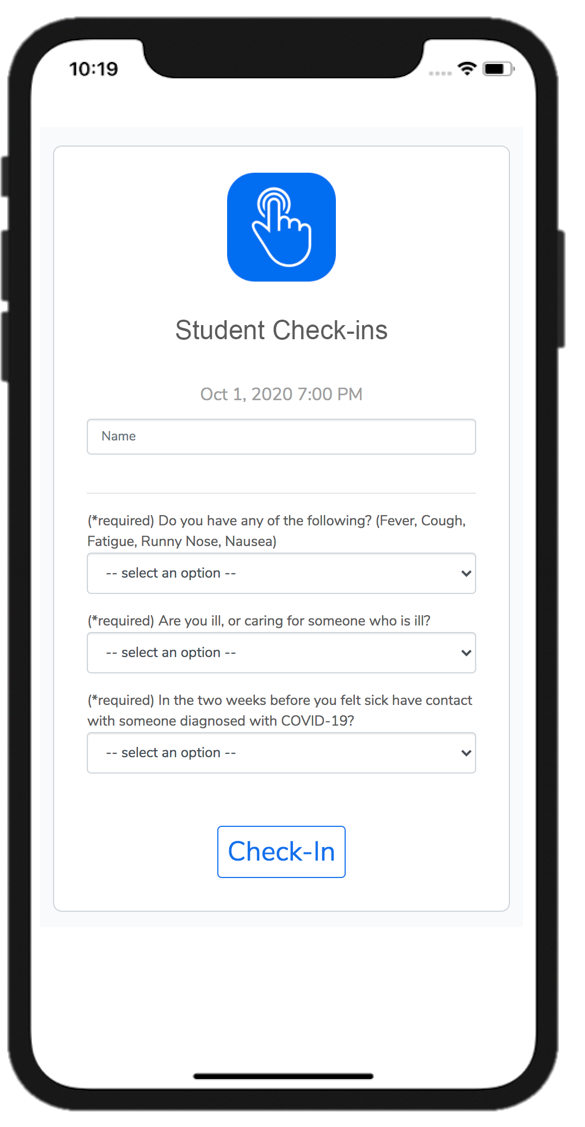A smartphone screen displaying a user interface for an app designed to manage student check-ins. Prominently featured in the middle of the screen is the heading "Student Check-Ins." Below this heading, a blue icon illustrates a finger surrounded by concentric circles, suggesting a focus on touch-enabled interaction. The displayed date and time read "October 1st, 7:27 p.m." Additionally, the interface includes text fields for inputting a student's name and selecting a health condition. An important section addresses COVID-19, inquiring about the illness status of the user or others. The design appears intuitive, aiming to streamline the process of recording student health information efficiently.